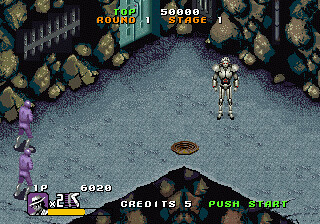This image is a detailed screenshot from a classic handheld or flash video game, set within a large, rocky room. The environment is marked by a textured gray floor, adorned in its center with a prominent bronze or brown circle. To the left, two characters clad in blue or purplish armor stand prepared. On the right side of the floor, another character in elaborate silver armor with red trim and a black outline takes position. Surrounding the central space, the rocky walls seem to be crumbling or in a state of decay, and between the rocks can be seen a fence-like structure, resembling a white picket fence but rendered in gray. Notably, there's a blue door positioned in the background.

Text overlays for gameplay are present: at the top center, "TOP" is written in green, followed by "ROUND" in orange next to "1" in black or white, accompanied by "50,000." Below this text, on one side, "STAGE" is displayed in orange and on the opposite side "1" in white, suggesting early game progress. Additional game information is provided at the bottom, indicating one player, five credits, and the current score. Overall, the scene encapsulates the nostalgic essence of classic arcade gaming.